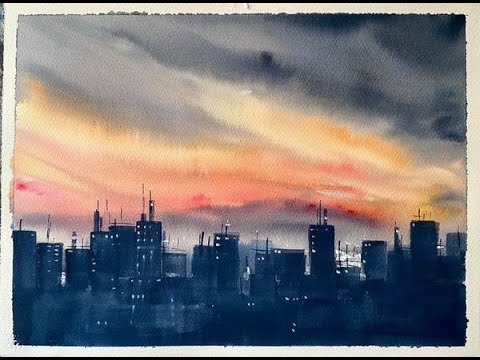The painting is a detailed depiction of a city skyline, prominently featuring tall buildings. The sky occupies the top portion of the painting, transitioning from nearly black, gloomy clouds at the top to vibrant hues of orange and pink as it descends, suggesting either a sunrise or sunset. The skyline itself reveals numerous high-rise buildings, many around 20-30 stories tall, adorned with antennas and dotted with white specks that represent illuminated windows. A smoky, industrial atmosphere envelops the buildings, hinting at an older, potentially aging city with a dark but not overwhelmingly menacing ambiance. Despite the lack of any text or specific markers indicating the city's identity or the artist, the painting captures a compelling, stylistically realistic urban scene under a dramatic sky.